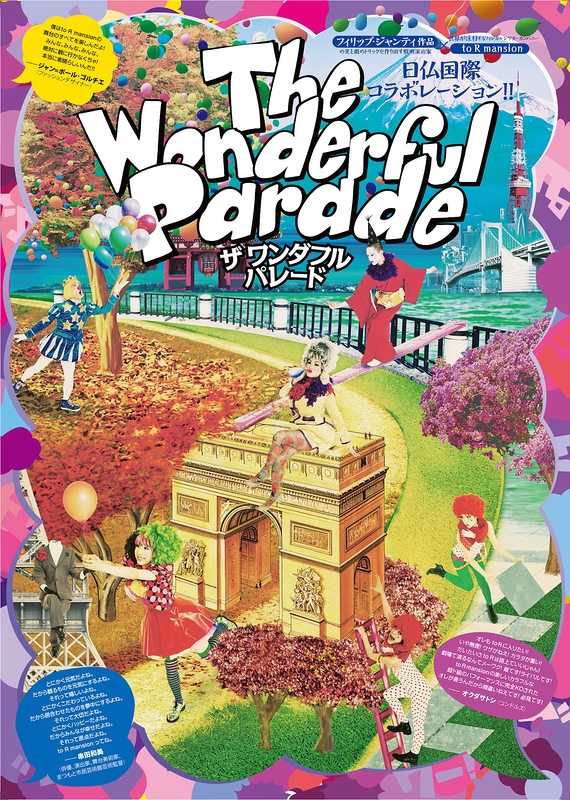The image is a vividly colorful poster titled "The Wonderful Parade" written in large, white puffy letters at the top center. Flanking the title is Asian script, with blue characters on the right and more Asian writing inside a yellow conversation bubble on the left. Below the title, the scene is bustling with activity and vibrant subjects, resembling a cross between an animated illustration and a paper doll setup.

The central scene features a yard with green grass, scattered leaves, trees, and a black fence. A white metal bridge, reminiscent of the Bay Bridge in San Francisco, spans the background with a boat passing underneath. A significant structure, akin to the Arc de Triomphe, but located by the coast with fencing and visible sea, is in the middle ground.

On this building, an Asian woman in a yellow dress sits perched at the top. Below her, another Asian woman walks across a long purple wooden beam that stretches from the fence to the roof of the building. The yard also hosts several other animated figures: one woman in a red dress, another in a white and red polka dot jumpsuit climbing a ladder, and a girl in a red hat and green leggings running from the grass to the pavement.

Balloon elements add to the festivity; a person holding balloons stands on leaves under a tree. Additionally, the lower corners of the poster feature conversation bubbles— a purple one with white Asian writing on the bottom right, and a blue one with white Asian writing on the bottom left.

Overall, the poster is strikingly detailed and lively, filled with an eclectic mix of animated figures, colorful elements, and a harmony of whimsical details and architectural backdrops.